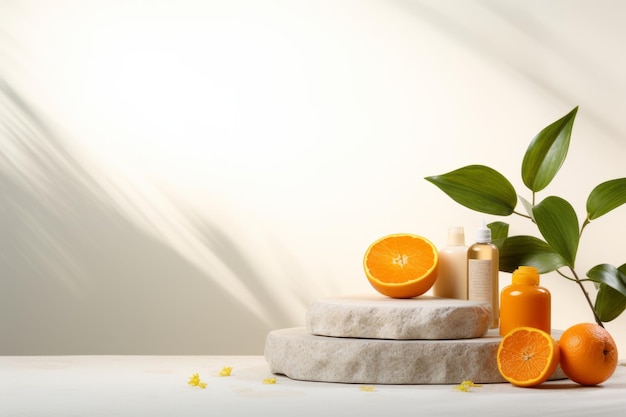In a minimalist white setting, this photographic still life features a collection of citrus fruits and skincare items arranged on a white counter with a subtle texture. Two stacked marble slabs serve as a stage for three unlabeled bottles—one filled with a vibrant orange substance, another with a clear liquid, and the third containing a white opaque cream or lotion, each capped with white tops. A whole orange and two orange halves, one of which appears to have been partially squeezed with some orange petals scattered in front, accompany the bottles. Additionally, a green leafy branch leans against the bottles, adding a touch of natural elegance to the composition. Shadows on the white background enhance the clean, serene atmosphere.